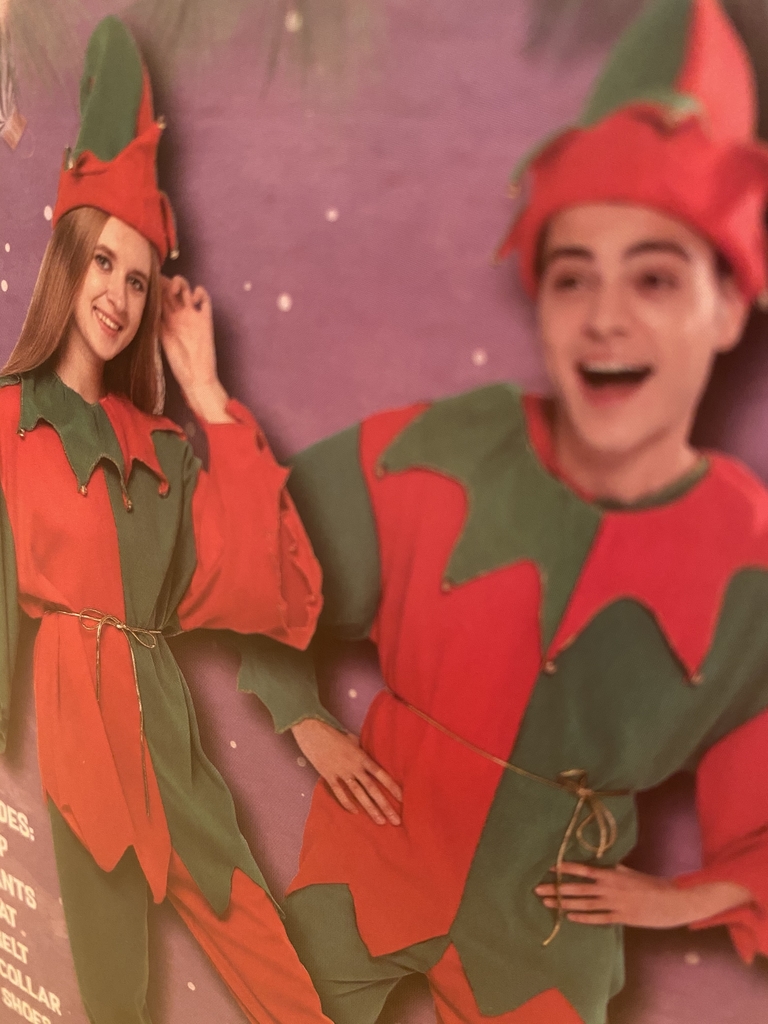This image captures the packaging of a costume featuring two children dressed as elves. On the left side, a girl with brown hair, partly brushed out of her face, stands as the main focus. She is smiling and wearing a red and green elf outfit with alternating colors—a red sleeve on one side and a green sleeve on the other, mirrored by her pants. The colors also alternate on her collar and elf hat, which is adorned with small brass bells. A gold rope belt cinches the outfit at her waist. To her right, a boy with darker hair and an excited expression, his mouth open, is dressed identically. Though he appears closer to the camera, he is more blurry, making him seem part of the background. Both costumes are detailed with alternating red and green sections and accessorized with gold belts and bell-decorated collars and hats. There is some unreadable text in the image's left corner.